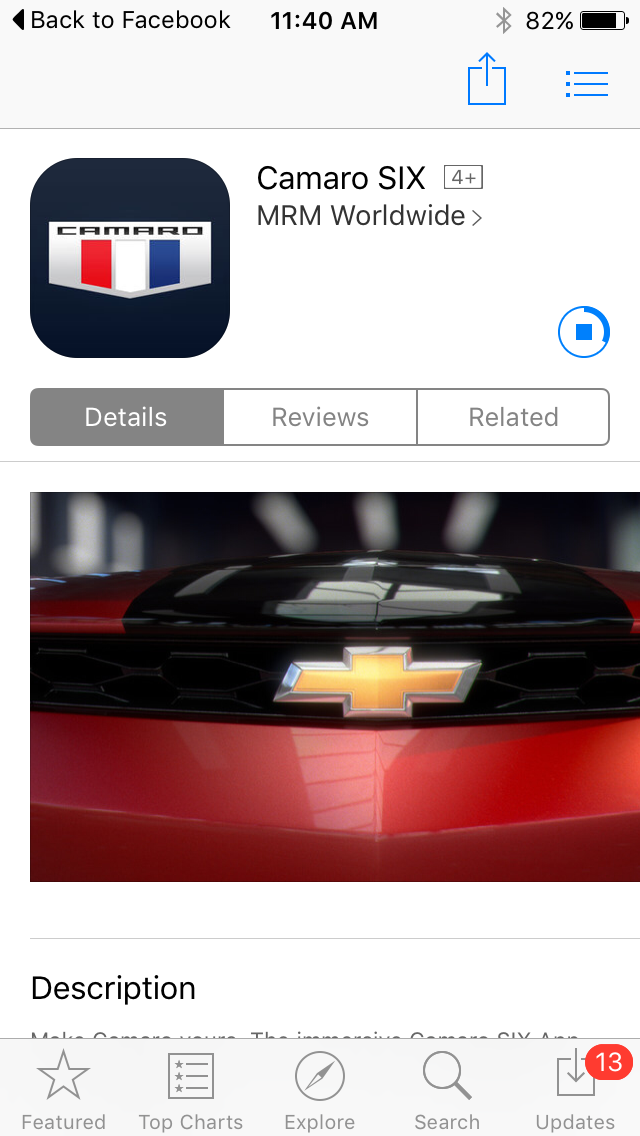This image appears to be a screenshot from a cell phone or an iPad, capturing an old version of the Apple App Store. The overall layout is rectangular and taller than it is wide. At the top, a light gray header hosts several icons and information: in the upper left-hand corner, a black arrow button labeled "Back to Facebook," indicating the user navigated from Facebook to the App Store. Centrally, the header shows the time, "1140 AM," while the upper right corner features a gray Bluetooth symbol and a battery icon showing 82%.

Beneath the header, there's a blue outline of the upload symbol, leading into the main content against a white background. On the left side, a black square with beveled edges prominently displays the shield logo for Camaro, featuring a red, white, and blue flag. To the right, the app's title "Camaro 6 MRM Worldwide" is clearly visible. Below this title, three navigation tabs are present: "Details" (highlighted), "Reviews," and "Related."

A rectangular photograph of a red and black Chevrolet Camaro follows, showcasing the car with a close-up of the yellow Camaro symbol, though finer details of the vehicle remain indistinct due to the close-up nature of the image. Below the photograph, the word "Description" marks the beginning of the app's info section.

At the very bottom, the footer displays several navigation icons: a star labeled "Featured," a piece of paper for "Top Charts," a compass icon with "Explore," a magnifying glass for "Search," and finally, "Updates" with a red circle indicating 13 pending updates. The overall aesthetic and elements suggest a rudimentary, earlier version of the App Store interface.